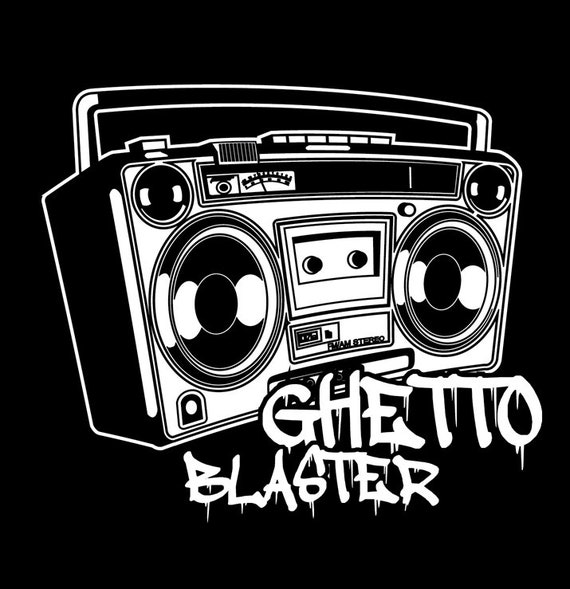The image is a detailed black and white digital drawing of an old-fashioned boombox, often referred to as a "Ghetto Blaster." At the very center of the image, the boombox, shaped like a horizontal rectangle, prominently displays two large speakers, one on each side. In the middle of these speakers sits the cassette deck with visible reels. On the top surface of the boombox, there are five push buttons, and adjacent to these are the radio dials. The boombox also features a large handle stretching across the top from one side to the other. Below the boombox, in dripping white lettering reminiscent of a spray-paint font, the words "Ghetto Blaster" are prominently displayed. The entire graphic sits against a plain black background, emphasizing the stark contrast and retro design of the boombox.